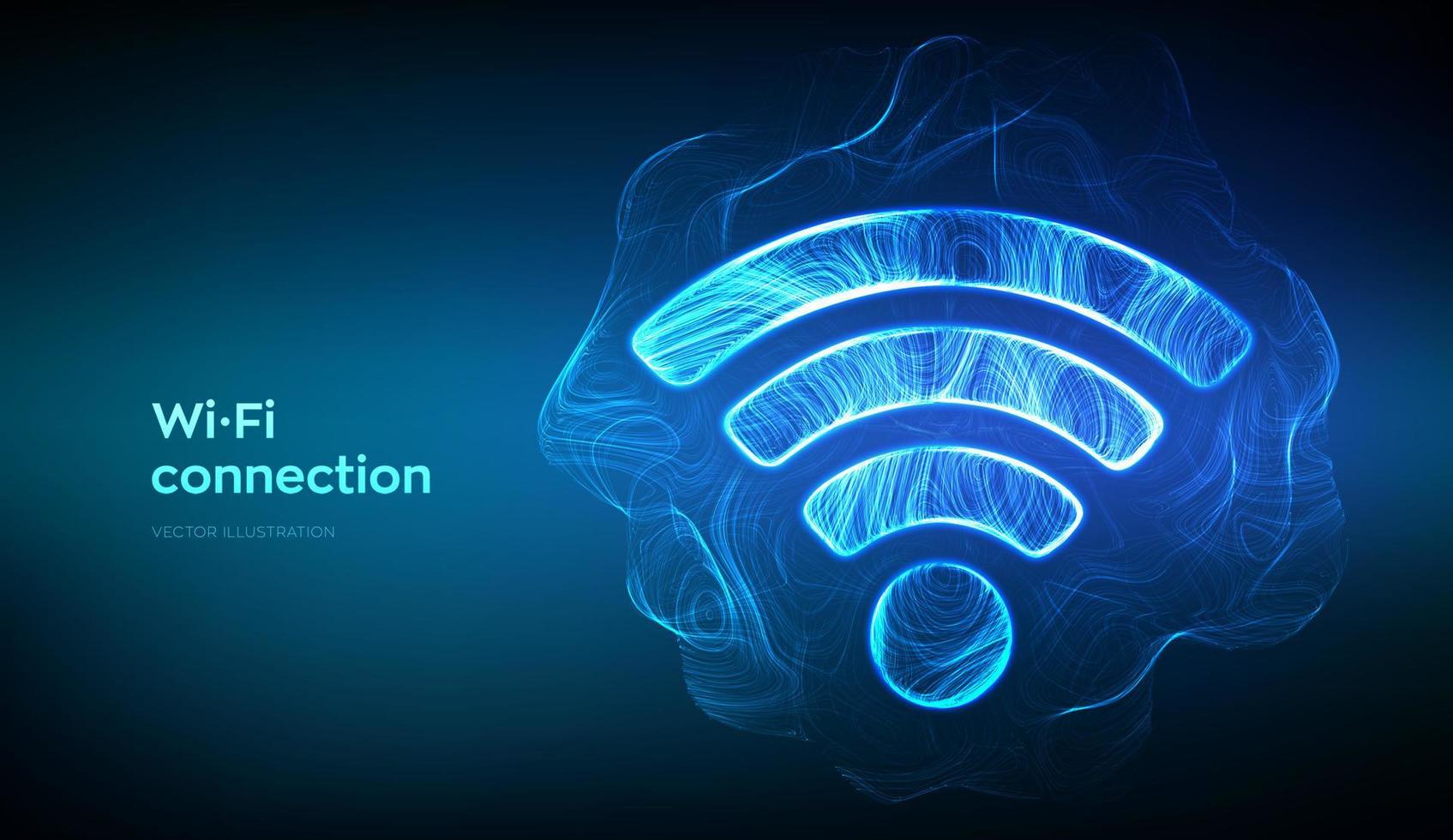This rectangular image features a Wi-Fi Connection Vector Illustration. The background has a gradient that transitions from an almost black dark blue at the edges to a slightly lighter, but still dark blue, towards the center. On the left side of the image, the text "Wi-Fi Connection" is displayed in a light blue or light greenish-blue color. Dominating the right half of the image is a bright blue Wi-Fi symbol composed of three arcs that increase in size as they move outward from a blue circle at the bottom. Surrounding the Wi-Fi symbol are wavy, cloud-like lines in shades of dark and light blue, adding a sense of radiating frequency and movement. The overall composition creates a striking visual contrast against the dark background, emphasizing the neon blue elements of the Wi-Fi symbol.